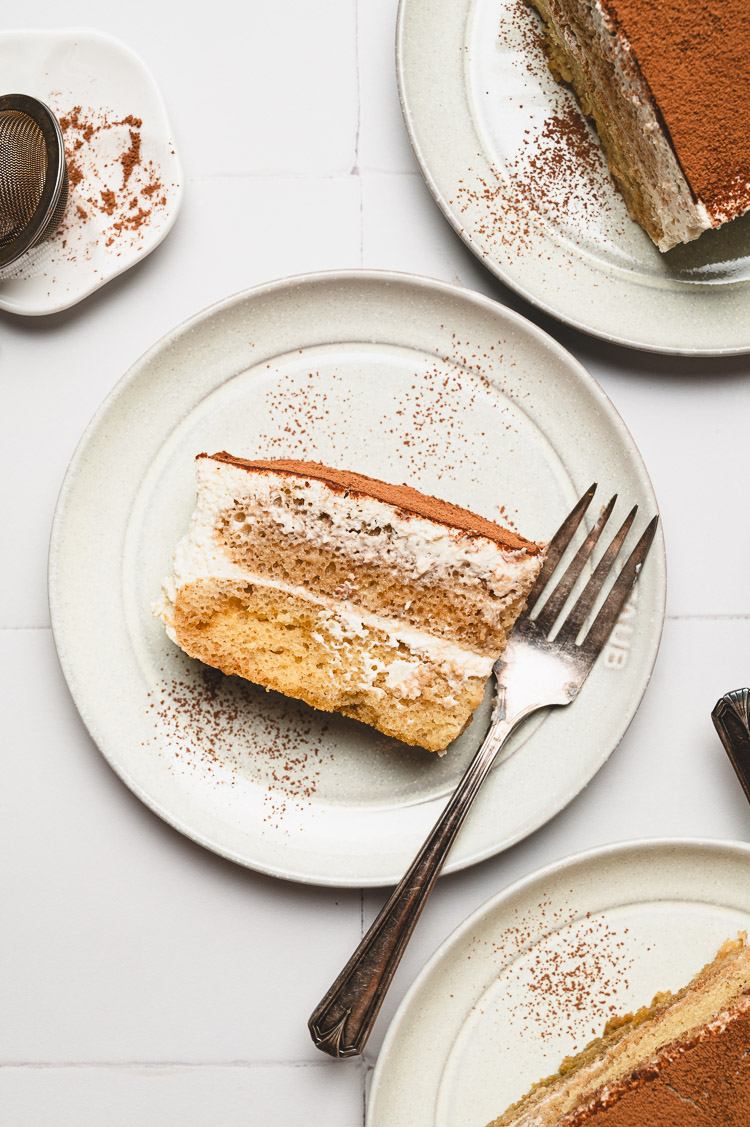The image showcases a meticulously arranged dessert setting on a white-tiled table, featuring multiple white plates of tiramisu. Dominating the center, a full plate presents a small slice of tiramisu, revealing its rich layers of dark brown cake, creamy white filling, and topped with a dusting of cocoa powder. A silver fork lies diagonally on this central plate, its tines pointing to the top right. Flanking this central composition, the top right and bottom right corners reveal partial glimpses of two more plates, each holding a larger, upright slice of tiramisu similarly dusted with cocoa powder. The scene is completed with a smaller, flower-shaped white plate in the top left corner, holding what appears to be a sieve, likely used to sprinkle the cocoa powder over the desserts. The overall arrangement highlights the intricate layers and textures of the tiramisu, evoking a sense of indulgent sophistication.